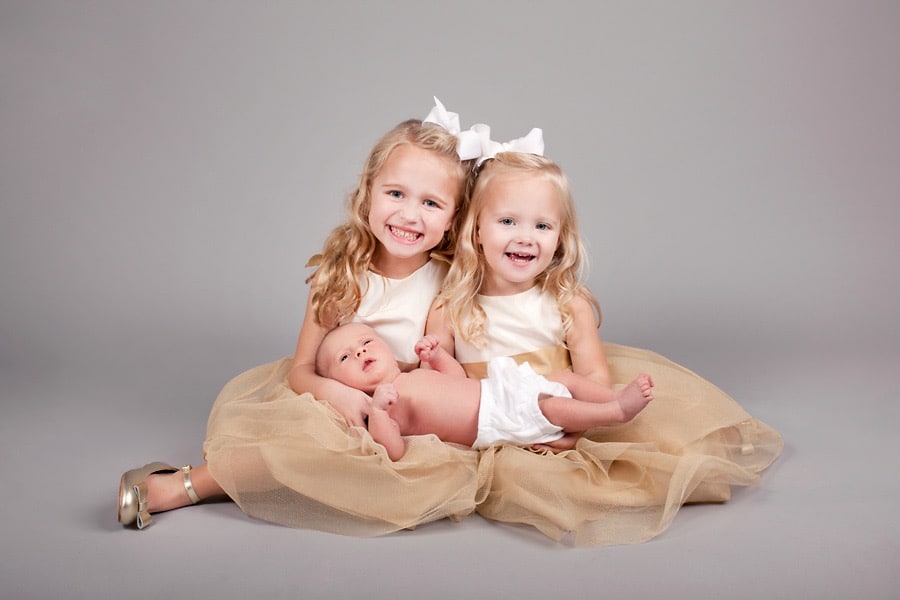This is a detailed photographic family portrait set indoors against a grey background, featuring three children. Two blonde girls, appearing to be around 3 or 4 years old and likely sisters, sit side by side with their heads close together. They are both smiling at the camera. The girls are dressed alike in sleeveless dresses with white tops and fluffy skirts—one description suggests the skirts are blue, while another says they are golden. Both girls have white bows in their hair and are wearing high silver shoes, though only one girl's shoes are visible as the other's feet are out of view. The girl on the right, slightly fairer in complexion, is missing some teeth, while the girl on the left has all her teeth. Spread across their laps is a baby in a white diaper, with short hair and arms raised as if in a bench-pressing position. The baby, whose gender is not discernible, is looking up towards the ceiling.